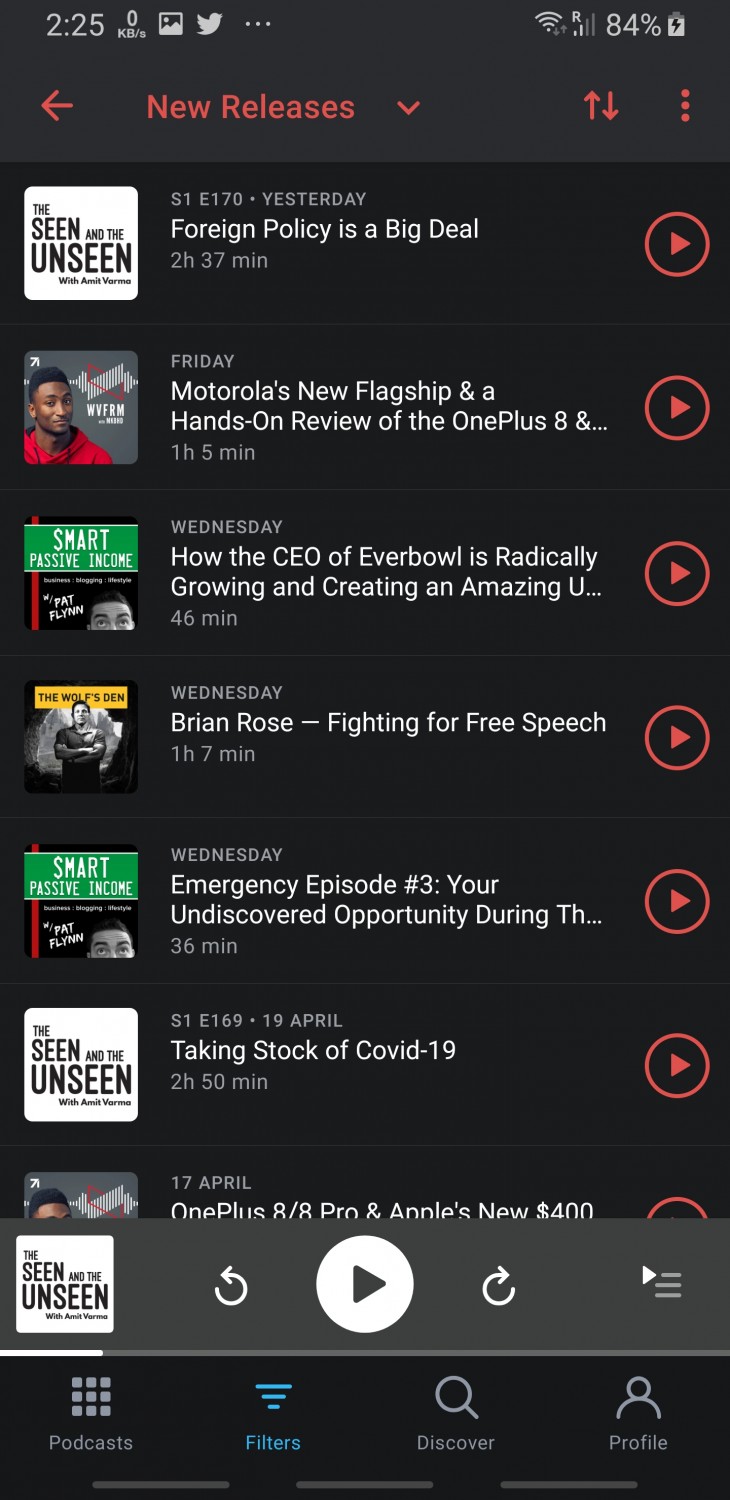This detailed screenshot captures the user interface of an Android-based music or podcast app, with the precise time marked at 2:25. Prominent indicators are present, including a download speed of 0 kilobytes per second in the top left corner, along with icons for pictures and Twitter, as well as a more options menu symbolized by three vertical dots.

The connectivity indicators show full Wi-Fi strength (3 out of 3), partial cellular signal (2 out of 4), and a battery level of 84%, actively charging. At the top of the interface, navigational elements include a back arrow and a drop-down menu labeled "New Releases," accompanied by sorting options and a menu symbolized by three horizontal bars.

The main section lists seven podcast options:

1. **Foreign Policy: It's a Big Deal (Season 1, Episode 170)**
   - *Time:* Yesterday
   - *Length:* 2 hours 37 minutes

2. **Motorola's New Flagship and Hands-on Review of the OnePlus 8**
   - *Release Date:* Friday
   - *Length:* 1 hour 5 minutes

3. **How the CEO of Everbowl is Radically Growing and Creating an Amazing You**
   - *Release Date:* Wednesday
   - *Length:* 46 minutes

4. **Brian Rose: Fighting for Free Speech**
   - *Release Date:* Wednesday
   - *Length:* 1 hour 7 minutes

5. **Emergency Episode #3: Your Undiscovered Opportunity During the...**
   - *Release Date:* Wednesday
   - *Length:* 36 minutes

6. **Taking Stock of COVID-19 (Season 1, Episode 169)**
   - *Release Date:* April 19th
   - *Length:* 2 hours 50 minutes

7. **OnePlus 8 / 8 Pro and Apple's New $400...**
   - *Release Date:* April 17th
   - Limited details provided.

Currently, "The Unseen" is being played, as shown by the playback bar at the bottom. The interface includes four main navigation areas: Podcasts, Filters, Discover, and Profile.